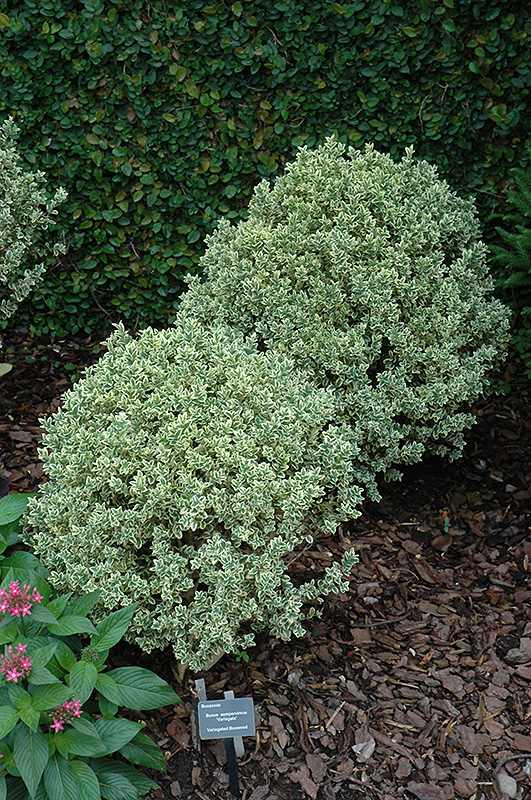This is a color photograph taken outdoors during the daytime, depicting a well-maintained garden area from a vantage point approximately six feet above the ground. The image features a close-up view of a flower bed covered with deep brown mulch. Dominating the foreground are two prominent shrubs characterized by lime green leaves that transition to a lighter, almost white hue at the tips. These shrubs are substantial in size and appear meticulously trimmed.

Adjacent to these shrubs, towards the left corner of the image, lies another flowering plant flaunting green leaves and delicate pink blossoms. A notable detail in the mulch is a black tag with white text, likely indicating the botanical names of the plants, hinting at a botanical park or garden setting.

In the background, filling the upper portion of the photograph, is a vast, dense hedge that forms a verdant green wall. This hedge also shows signs of recent trimming and meticulous upkeep, contributing to the overall impression of a well-tended and orderly garden space.